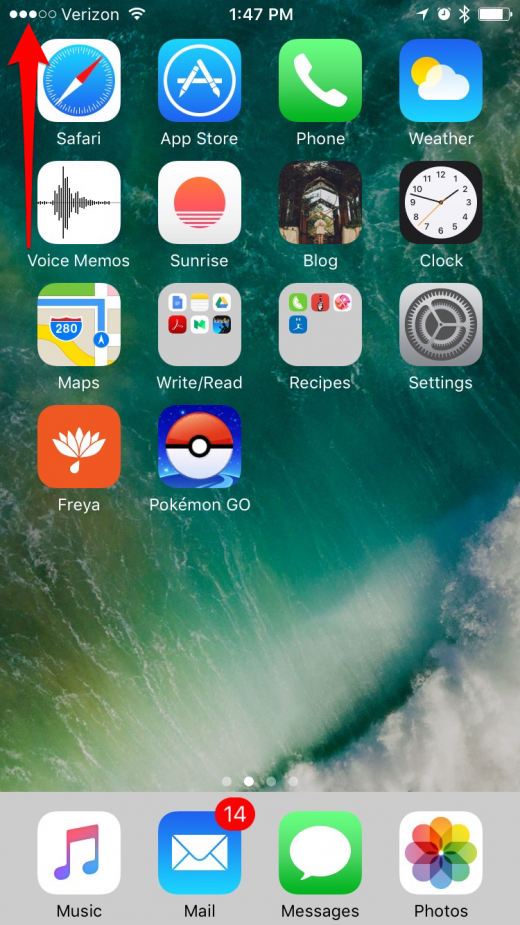This screenshot captures the home screen of a mobile device, specifically an iPhone. The top of the screen displays the typical status icons: the time, Wi-Fi connection, Bluetooth connection, and battery status, all providing quick reference information about the phone's current state. On the top left corner, there are three solid white circles aligned horizontally, next to which are two unfilled circles. A red arrow points upwards toward the three white circles, drawing attention to them.

The main portion of the screen showcases a familiar iPhone interface, complete with several app shortcuts. There are approximately 14 app icons present, including commonly used functions such as Maps, Pokémon GO, Weather, and the App Store. Additionally, there are a couple of folders, each containing multiple apps, labeled for activities like "Recipes" and "Read and Write," indicating an organized approach to app management.

At the bottom of the screen, the navigational menu features essential apps: Music, Mail, Messages, and Photos. The background of the home screen displays a stunning aerial view of the sea with waves, adding a serene and natural aesthetic to the digital interface.